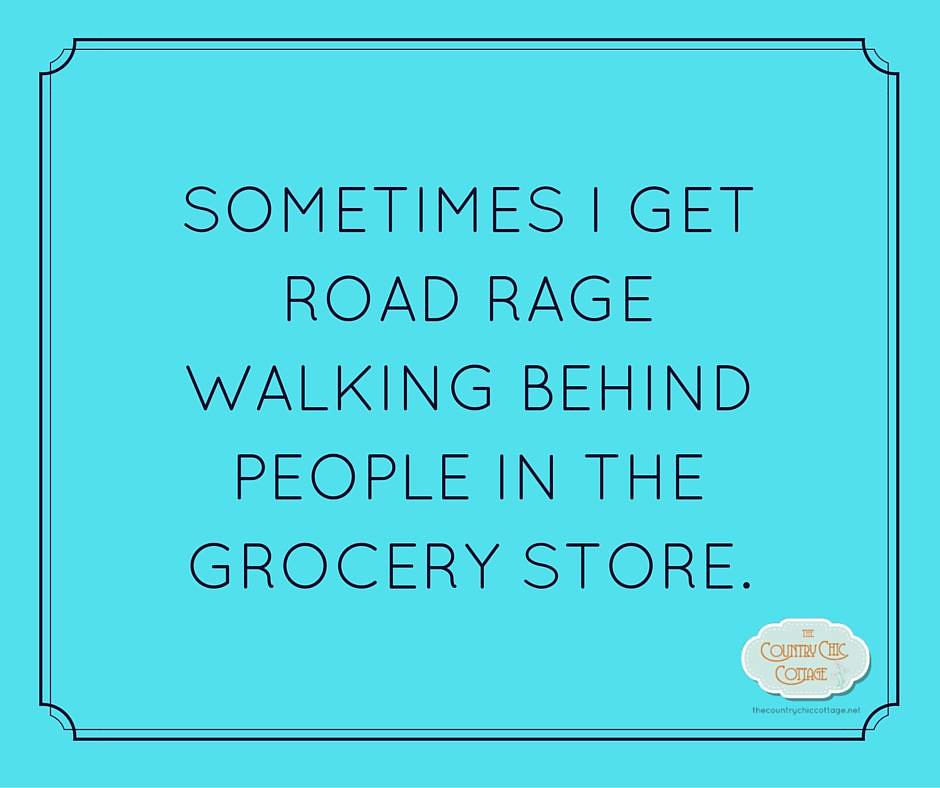The image is a horizontally rectangular graphic with a light pastel robin's egg blue background. It features a decorative black border, which consists of a combination of bold and thin lines with a slight decorative swoop in each of the corners. The text in the center is in black, all-capital letters, and reads: "Sometimes I get road rage walking behind people in the grocery store." In the lower left corner, there is a small whitish cloud-shaped logo that reads "The Country Chic Cottage" along with an accompanying website, though the URL is not clearly legible. The overall design is simple and resembles the style of an old person meme typically found on social media platforms like Facebook or Instagram.